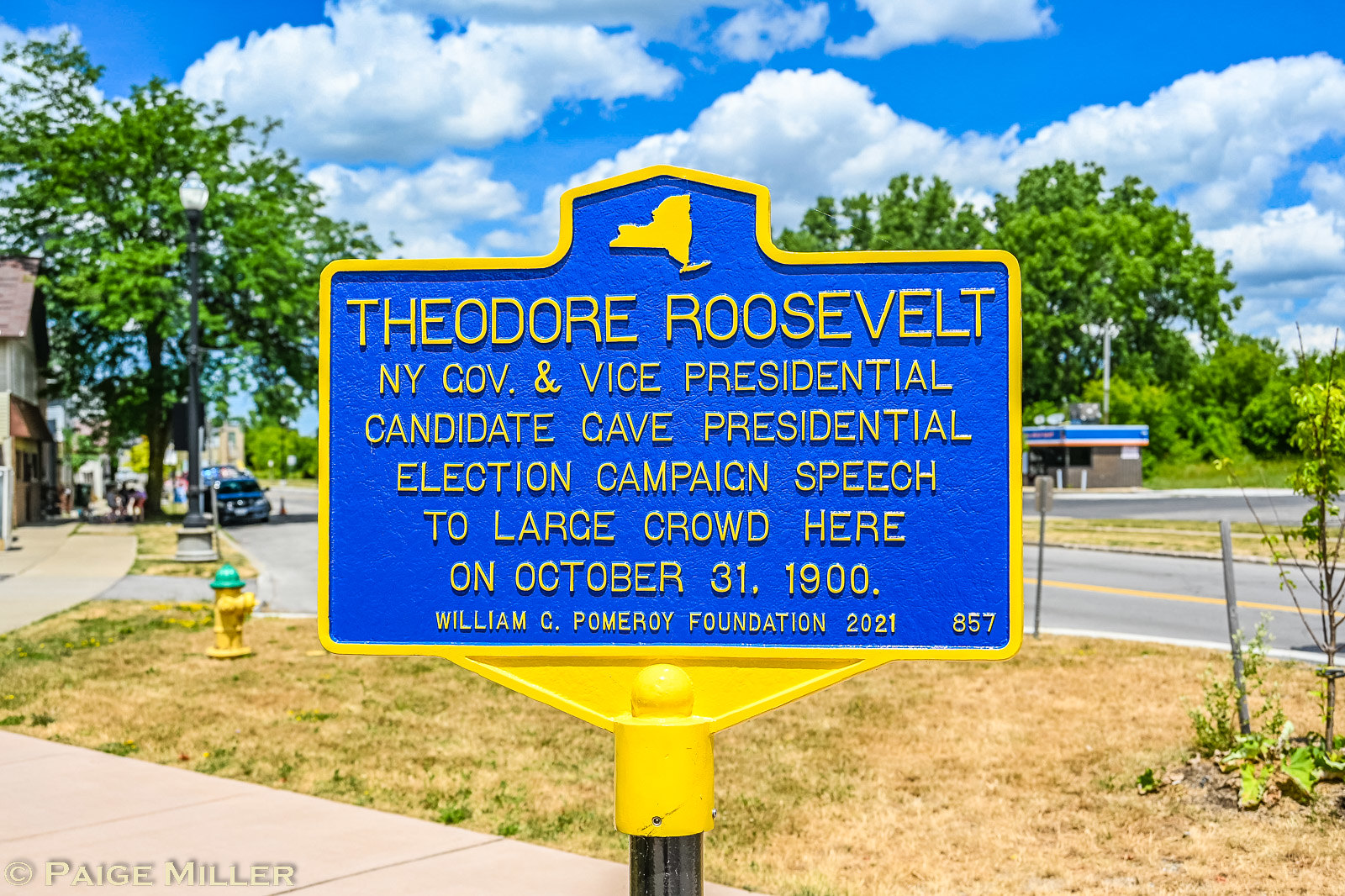The image depicts a historical marker set on a metal pole against an outdoor backdrop reminiscent of a residential area. The marker features a blue plate with gold borders and text, and at the top, an insignia of New York State. The sign reads: "Theodore Roosevelt, New York Governor and Vice Presidential Candidate, gave a Presidential Election Campaign Speech to a large crowd here on October 30th, 1900." The marker was established by the William C. Pomeroy Foundation in 2021, bearing the identifier 857. Beneath this, the name "Paige Miller" is visible, likely crediting the photographer. Surrounding the marker are elements of the neighborhood: brown grass, a yellow fire hydrant, scattered trees, and people walking in the distance. Across the street, partly observable, is what appears to be a gas station. The sky above is sunny with scattered cumulus clouds, lending a bright and clear atmosphere to the scene.